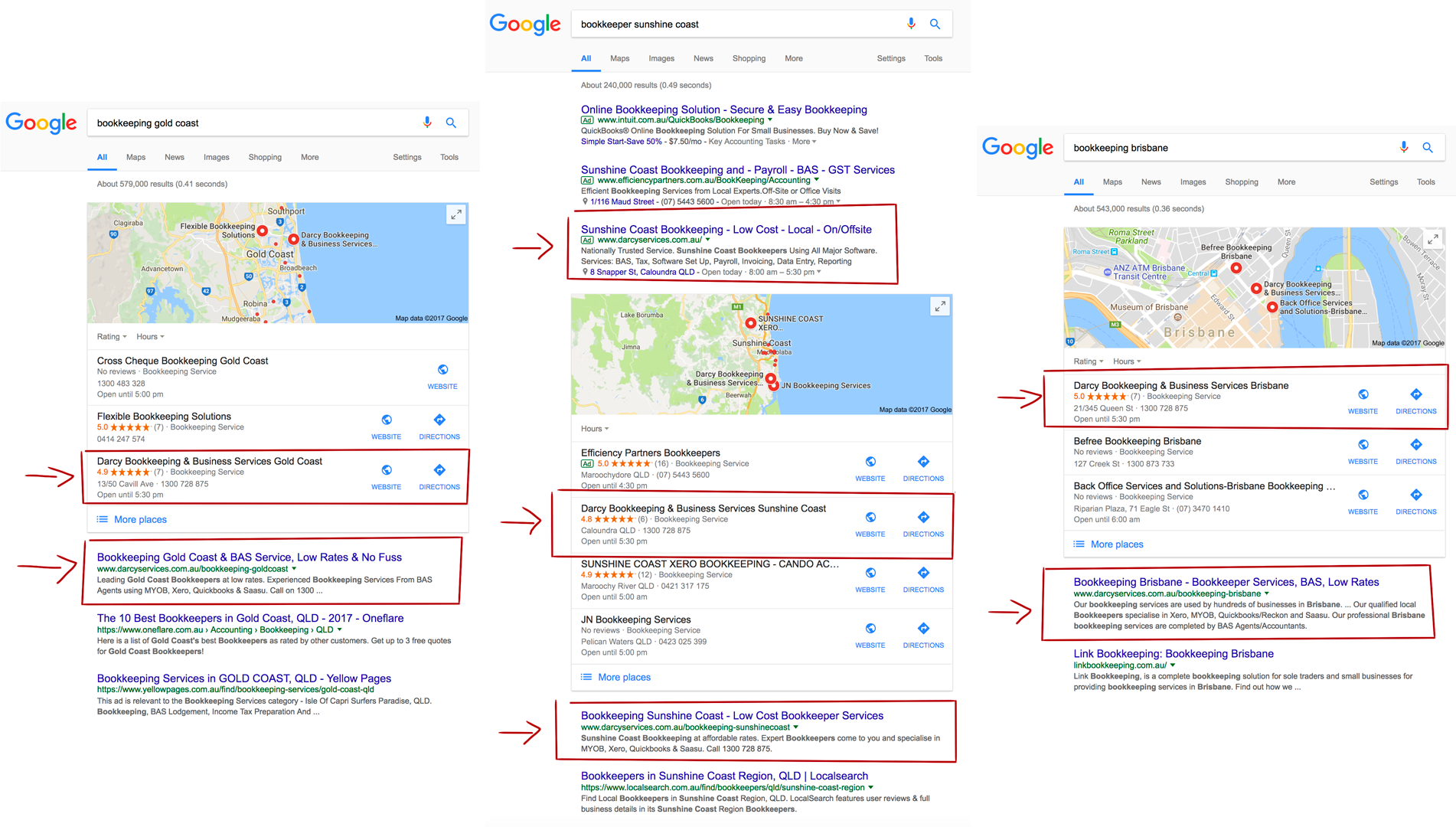The image consists of three side-by-side screenshots depicting Google search results for bookkeeping services in different Australian cities. 

- **Left Panel**: The search query is "bookkeeping Gold Coast." It features a map of the Gold Coast and highlights two specific businesses with a red rectangle. A red arrow points toward this rectangle for emphasis.

- **Middle Panel**: The search query changes to "bookkeeping Sunshine Coast." This panel displays more diverse search results. Three ads or search results are highlighted within a red rectangle, each indicated by a red arrow for clarity.

- **Right Panel**: The search query is "bookkeeping Brisbane." The results show that two specific businesses, "Darcy Bookkeeping" and "Bookkeeping Brisbane," appear in each of the three searches. This panel emphasizes the consistency of these businesses across different search locations, helping to illustrate their broad online presence and relevance.

This detailed comparative analysis aims to demonstrate the consistency and prominence of certain bookkeeping businesses across various regional searches.